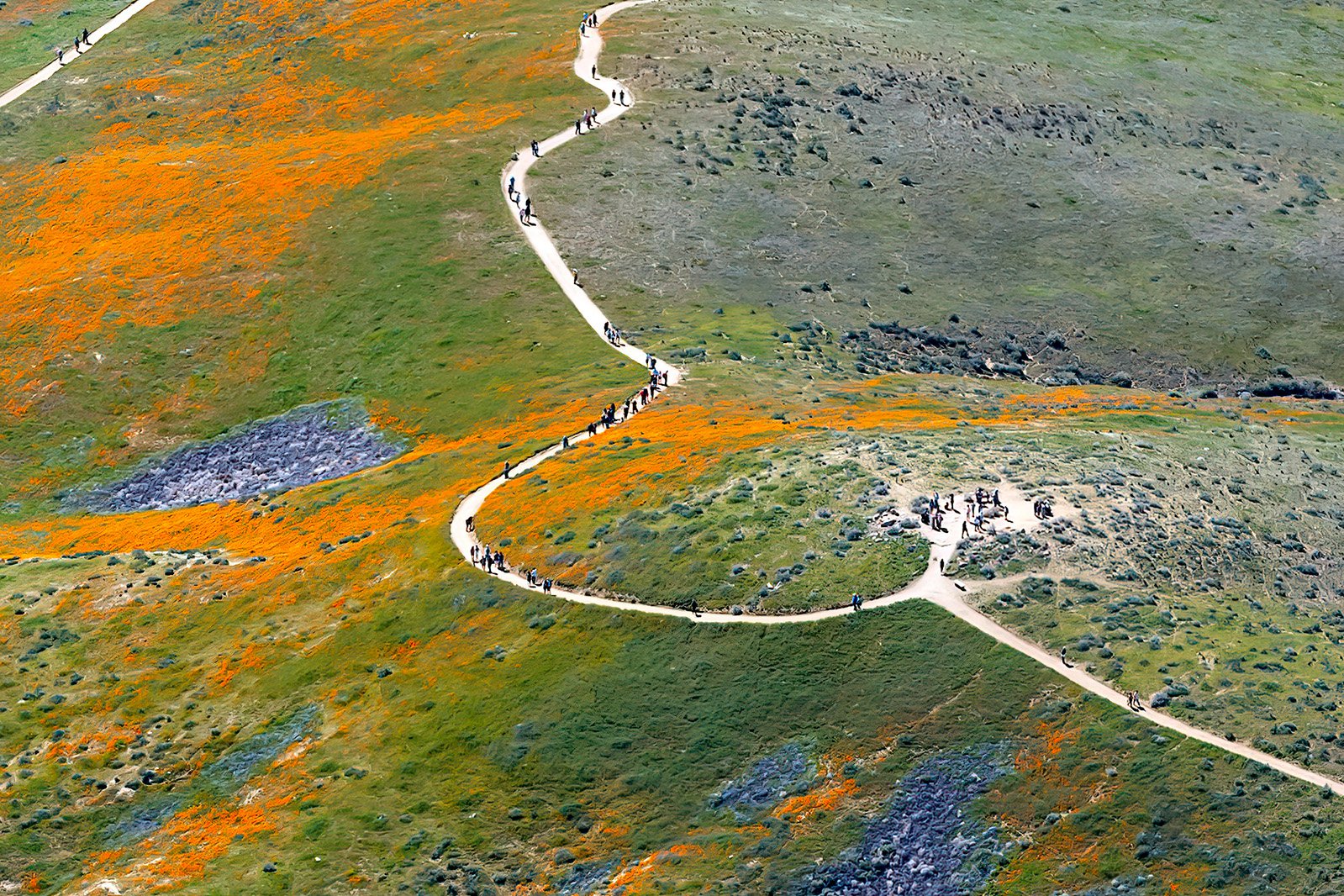This aerial image showcases a rolling landscape with gentle hills, characterized by a prominent paved or concrete pathway that meanders diagonally through the scene. Starting from the bottom right, the pathway zigzags up the hills, creating a semi-circular loop before continuing to a clearing at the top hill's summit and then extends onward. The landscape is a mosaic of vibrant green, orange, and gray hues. The green dominates the left hillside, indicative of lush grass, while patches of orange suggest seasonal grasses or perhaps flowers. The right hillside has a more barren, rocky appearance with areas of brown soil. Scattered across the image are rocks and people trekking along the walkway, with a notable gathering of 10 to 15 individuals at the hilltop clearing. The blue objects seen near the image's bottom right and left edges hint at manmade elements. The sunlight bathes the entire terrain, highlighting the diverse colors and textures of the landscape.